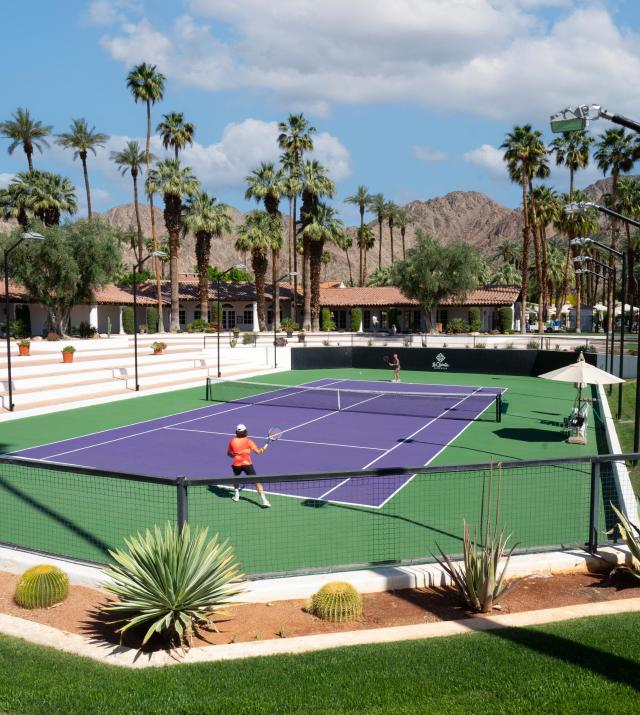The image showcases a vibrant tennis match set in a striking desert environment. At the center, there's a well-maintained tennis court with a distinctive purple playing surface bordered by a green outer edge. Two players are engaged in a match: the player in the foreground is wearing an orange shirt, and they appear to have just served the ball with their right hand. A second player can be seen on the opposite side of the court. The area features manicured green grass surrounding the court, which is enclosed by a green fence adorned with desert plants, including cactuses and other spiky flora.

On the left-hand side, there's a seating area with tiered steps, and an umbrella can be seen on the right. Taller lights frame the court, presumably for nighttime play, enhancing the setup's elegance and functionality. In the background, a clubhouse is visible, complemented by tall palm trees and additional desert plants. Farther in the distance, towering, jagged mountains rise against a backdrop of a blue sky dotted with puffy white clouds, adding depth to this picturesque scene. The overall impression suggests a high-end facility, possibly a resort or a country club, nestled in a valley that might be reminiscent of regions like California.